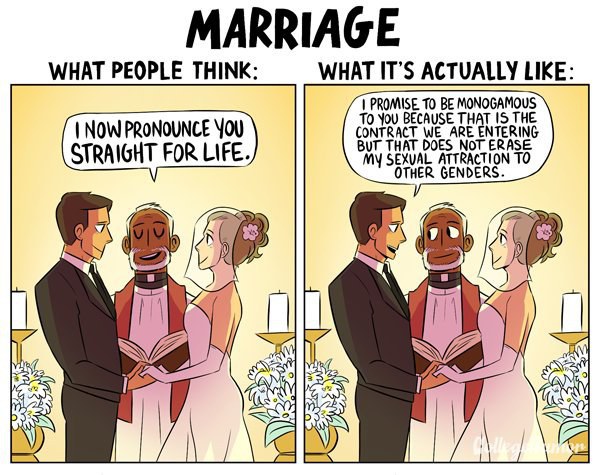The image is a satirical cartoon about marriage, with the title "MARRIAGE" prominently displayed at the top in capital letters. It is divided into two panels labeled "What People Think" on the left and "What It's Actually Like" on the right. 

In the left panel, under "What People Think," a man wearing a brown suit is holding hands with a woman in a white bridal dress, complete with white gloves, a transparent veil, and a flower in her hair. An African American priest, with his eyes closed, holds a book and stands in the middle, while candles and flowers flank the altar on either side. The priest declares, "I now pronounce you straight for life."

The right panel, under "What It's Actually Like," mirrors the scene with subtle differences. The man in the brown suit now has his mouth open, while the priest has his eyes wide open, looking at him. The priest says, "I promise to be monogamous to you because that is the contract we are entering, but that does not erase my sexual attraction to other genders." The same candles and flowers adorn the altar as in the left panel, tying both scenes together.

The overall cartoon employs humor to comment on the complexities of marital commitment and societal expectations, highlighting that getting married does not change one's inherent sexual attractions. The image features a lighthearted, yet pointed, critique of conventional views on marriage.